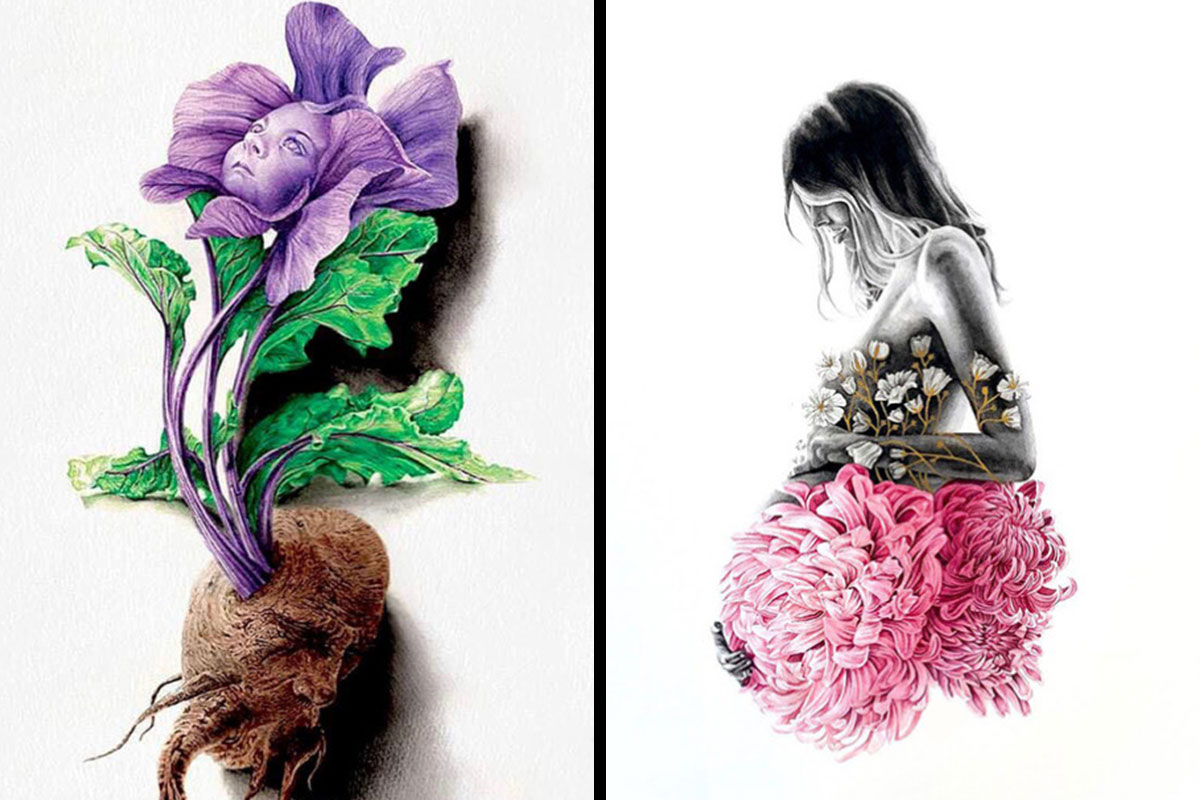The image consists of two computer-generated illustrations set side-by-side, creating a single, unified, fantasy-themed scene. Divided by a black vertical line, the left illustration features a surreal, purple-flowered plant emerging from a large brown root ball. The plant has dark green leaves beneath its light lavender petals, and the stem is also purple. Uniquely, where the flower's bud would be, there is a slightly eerie baby face, sharing the flower's lavender hue and looking upwards. This face is nestled among the petals, blending seamlessly with the blossom.

On the right side, the illustration depicts a black and white profile of a woman. She has long hair that partially obscures her face and is looking downward. Her upper body is intricately wrapped in white flowers and vines, reminiscent of tulips, which entwine her arms and chest. Her right hand cradles her belly, which transforms into cascading clusters of pink, seaweed-like leaves that drape down her midsection. The woman's figure is distinct and stylized, contrasting the more vivid and fantastical floral elements. Both illustrations share a white background, enhancing the detail and colors of the elements within.